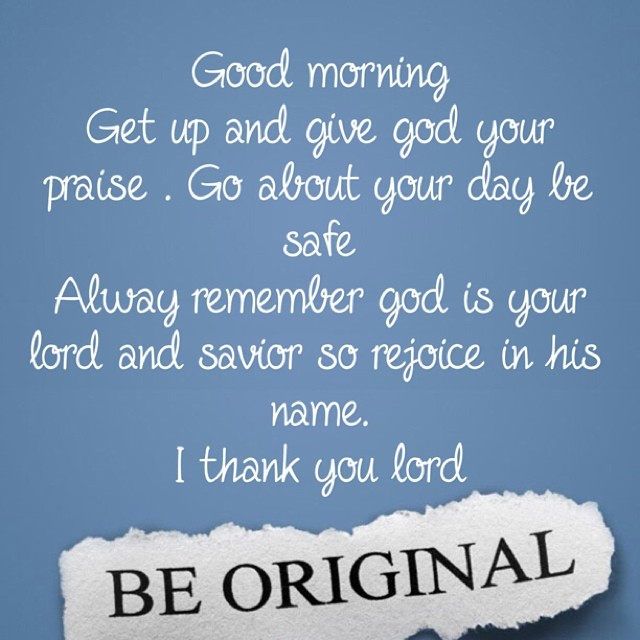The image features a light blue background with a series of motivational messages written in white, cursive text. At the top, it begins with "Good Morning," followed by a sequence of centered phrases: "Get Up and Give God Your Praise," "Go About Your Day, Be Safe," and "Always Remember God Is Your Lord and Savior, So Rejoice in His Name." Towards the bottom, the message concludes with "I Thank You, Lord." Beneath this text, there is a torn piece of paper layered on the image, displaying the words "Be Original" in black letters against a white background. The overall presentation emphasizes the importance of faith, safety, and originality.